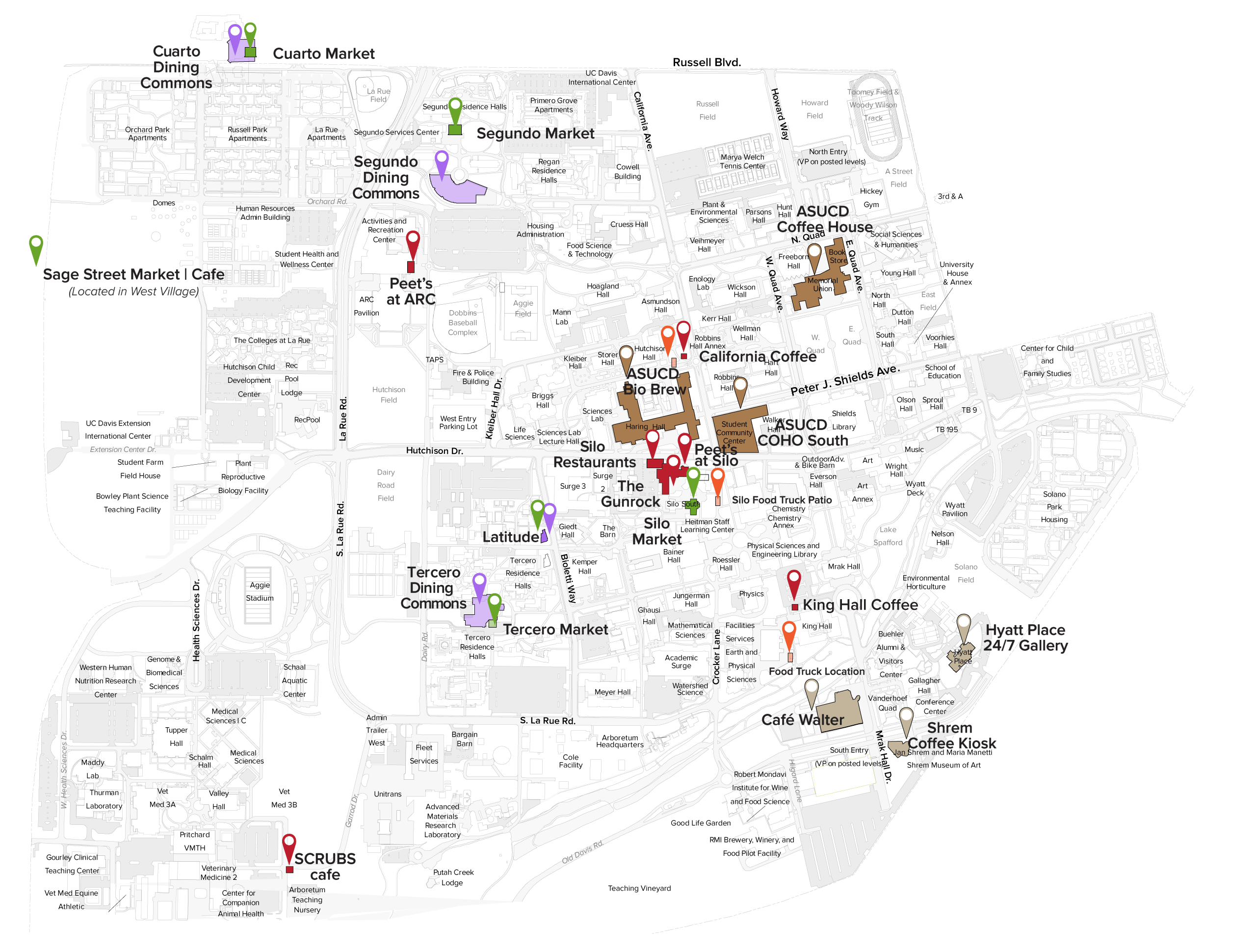This image depicts a detailed black and white map of a location, possibly the University of California, Davis (UC Davis), featuring a network of gray grid lines representing streets and buildings, with various landmarks highlighted and labeled with small text. The fonts vary in size, making some difficult to read, yet notable locations such as the ASUCD (Associated Students, University of California, Davis) Coffeehouse, the Segundo Market, and the Cuarto Market are marked prominently. 

Colored location pins enhance the map's readability, each color visualizing different types of sites: red pins indicate dining locations, brown pins highlight coffeehouses or drink establishments including the ASUCD Coffeehouse, ASUCD BioBrew, and ASUCD Coho South, green pins mark markets, purple pins designate commons like the Tercero Dining Commons, and orange pins signify food trucks. Other labels include the California Coffee, Cafe Walter, Shrem Coffee Kiosk, Hayah Place, and the 24-7 Gallery, indicating a diverse range of amenities and facilities across the mapped area.